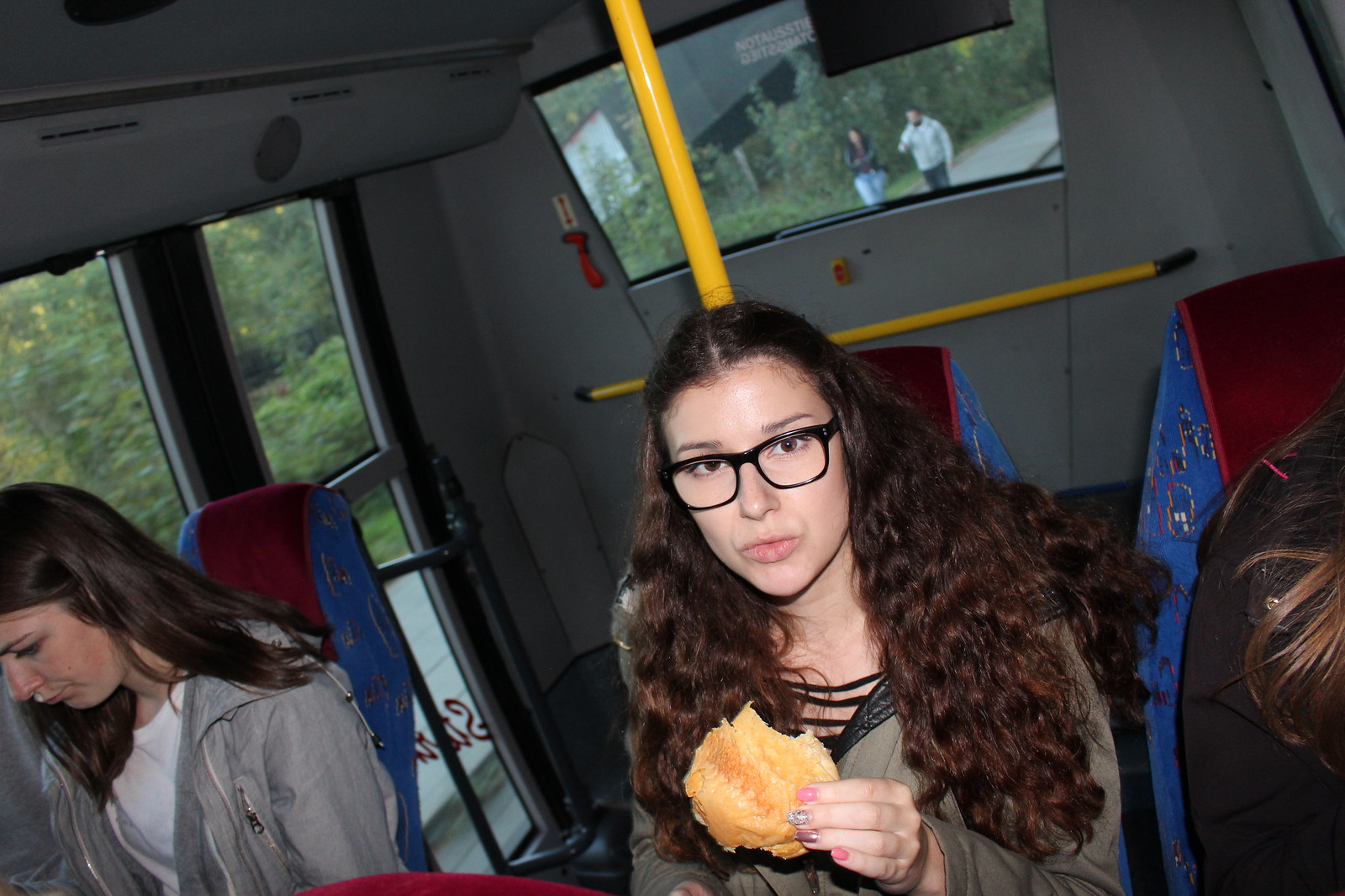The photograph captures what seems to be a spontaneous moment on a bus featuring a young woman with fair skin sitting in the center of the frame. She has long, wavy, brown hair and wears distinct, thick black-rimmed glasses. Her nails are painted in various glittery colors, including pink, silver, and purple. She is in the middle of eating a pastry, possibly a croissant or a danish, with a visible bite taken out of it, and she doesn't appear particularly pleased to be photographed. She is dressed in a green hoodie or jacket and sits on a red-backed, blue-sided seat. 

To her immediate left is another young woman with similar brown hair, clad in a white T-shirt and a gray jacket, who appears to be engrossed in something unseen, possibly an iPad or a book. To the right, barely in the frame, is an individual with long, dark hair and a black shirt. Yellow safety poles are noticeable in the bus; one is vertical directly behind the central figure, and another horizontal one is visible at the back of the bus. 

Through the back window, outside, the lush greenery of trees and bushes can be seen, along with two people walking on the pavement—a man in a white top and dark pants, and a woman in a dark top and white pants.